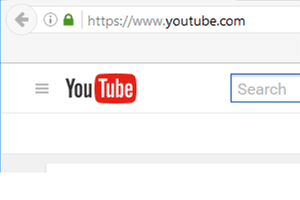This image is a highly zoomed-in screenshot of the YouTube website. The background is a mix of gray and white, contrasting against various interface elements. On the left side, adjacent to the URL, there is a green padlock icon indicating a secure connection, followed by an information button symbol. Next to the padlock and information button stands the URL text field, displaying the website address, "https://www.youtube.com." To the left of the URL, there's a back button, suggesting navigation capabilities.

In the middle left part of the screenshot, a portion of the YouTube logo is visible. The letters "You" are displayed in black, while "Tube" features white lettering inside a red rectangular button outline. Towards the right side of this logo section, there's a search bar bordered in blue, awaiting user input. The overall environment is typical of YouTube's interface, but the zoom level makes it appear fragmented and focuses on these specific elements.